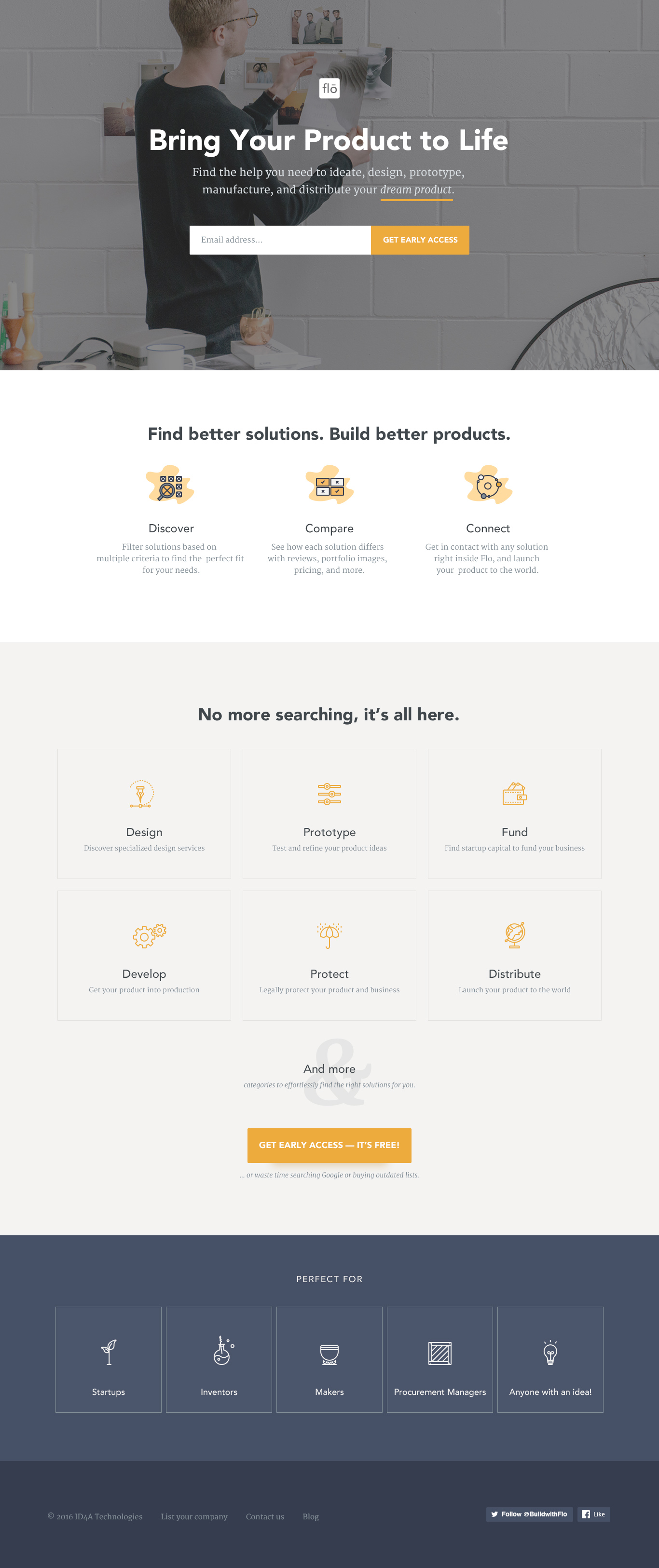A detailed and descriptive caption for the image:

This is a template for an app designed to guide users through the process of bringing a product to market. At the top of the template, there's a prominent hero image featuring a slender Caucasian man with short blonde hair and glasses, taping photographs to a white painted cinder block wall. He is wearing a blue long-sleeve shirt. Overlaying this image is the motivational headline "Bring Your Products to Life," although the original voice note mentioned "Light" by mistake. Central to the interface is the app's "FLO" icon, situated below a logo, along with the tagline, "Find the help you need to ideate, design, prototype, manufacture, and distribute your dream product." The phrase "Dream product" is underlined in yellow for emphasis.

Adjacent to this central area is an orange call-to-action button labeled "Sign Up, Get Early Access," alongside an email address input field, both encapsulated within the same rectangular space.

Further down, the template emphasizes user engagement with a section titled "Find Better Solutions, Build Better Products." This section includes three interactive options: Discover, Compare, and Connect, each accompanied by graphic icons with amoeba-shaped backgrounds.

Beneath this is a declaration, "No more searching, it's all here," followed by six more icons and sections arranged in a three-by-two grid. These sections are labeled as Design (featuring a light bulb icon), Prototype, Fund (with a wallet icon), Overlap, Protect (represented by an umbrella icon), and Distribute.

Towards the bottom of the template, there's a call to "Fund More & Get Early Access," accentuated by a yellow button labeled "It's Free." The segment highlights that the app is perfect for startups, inventors, makers, procurement managers, and anyone with an idea. These user categories are displayed within bordered squares set against a light slate blue background.

Finally, the footer contains additional information which is too small to be legible in the provided description.